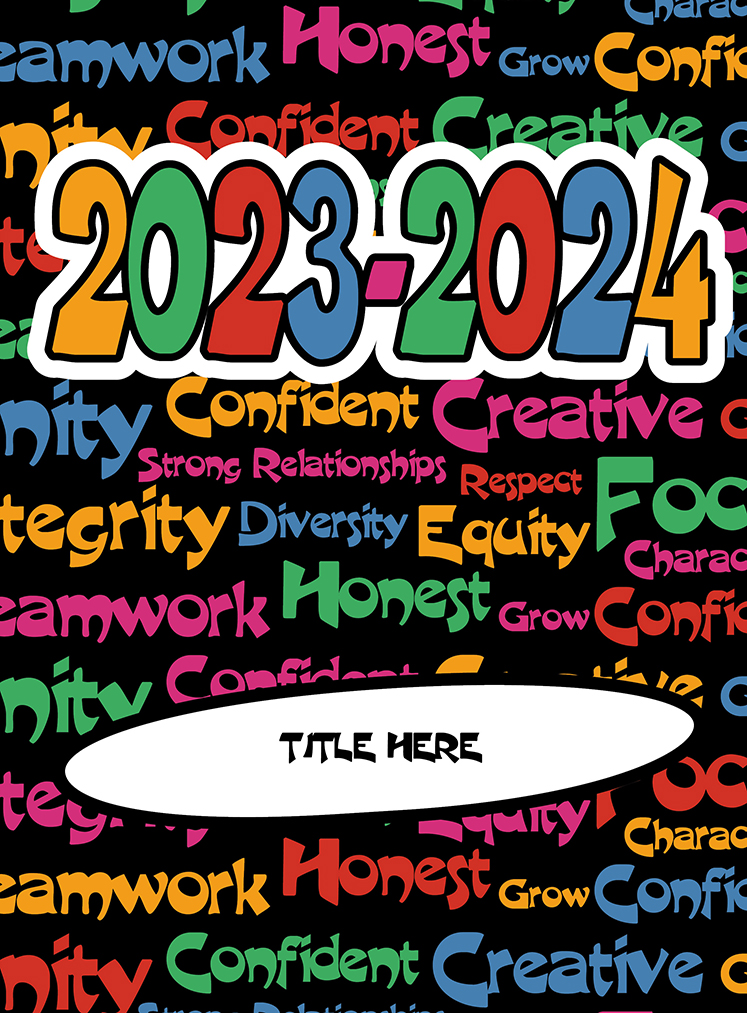This vibrant and motivational illustration, which could be fitting for the front of a diary, book, or poster, features a black background adorned with empowering words like "teamwork," "honest," "grow," "confident," "creative," "respect," "equity," and "diversity" in a modern, funky text. The colorful typography includes shades of blue, red, pink, green, and yellow, creating dynamic rows across the canvas. Prominently displayed in the center, the years "2023-2024" stand out with a chunky cloud-like white outline around multicolored numbers: a yellow 2, green 0, red 2, blue 3, pink dash, green 2, red 0, blue 2, and yellow 4, each digit outlined in black. At the bottom third of the illustration lies an elongated oval bubble with a black outline and white fill, containing the placeholder text "TITLE HERE" in bold, capitalized black letters. This detailed and colorful design brings an energetic and optimistic feel, making it perfect for motivating and inspiring those who view it.